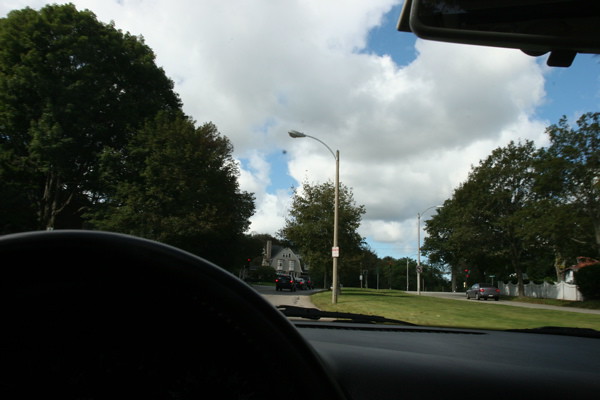This photograph offers a point-of-view perspective from the driver’s seat of a vehicle, giving a detailed view of the black dashboard, steering wheel, and wiper blade. Visible through the windshield, a lush green median separates two lanes of traffic, each bordered by dark green oak trees with dense leaves and a few street poles. Directly ahead, two vehicles occupy the same lane as the driver, while another small vehicle is visible across the median. On the opposite side, a black truck with its brake lights illuminated is positioned in front of a gray, two-story house. Additional details include a white house with a parked car in front of it, a low-hanging tree, and a strip of grass running between the roads. The sky above is a mix of blue patches and large, white clouds, contributing to an overall clear day. A portion of the rearview mirror is also visible in the top right corner of the image.